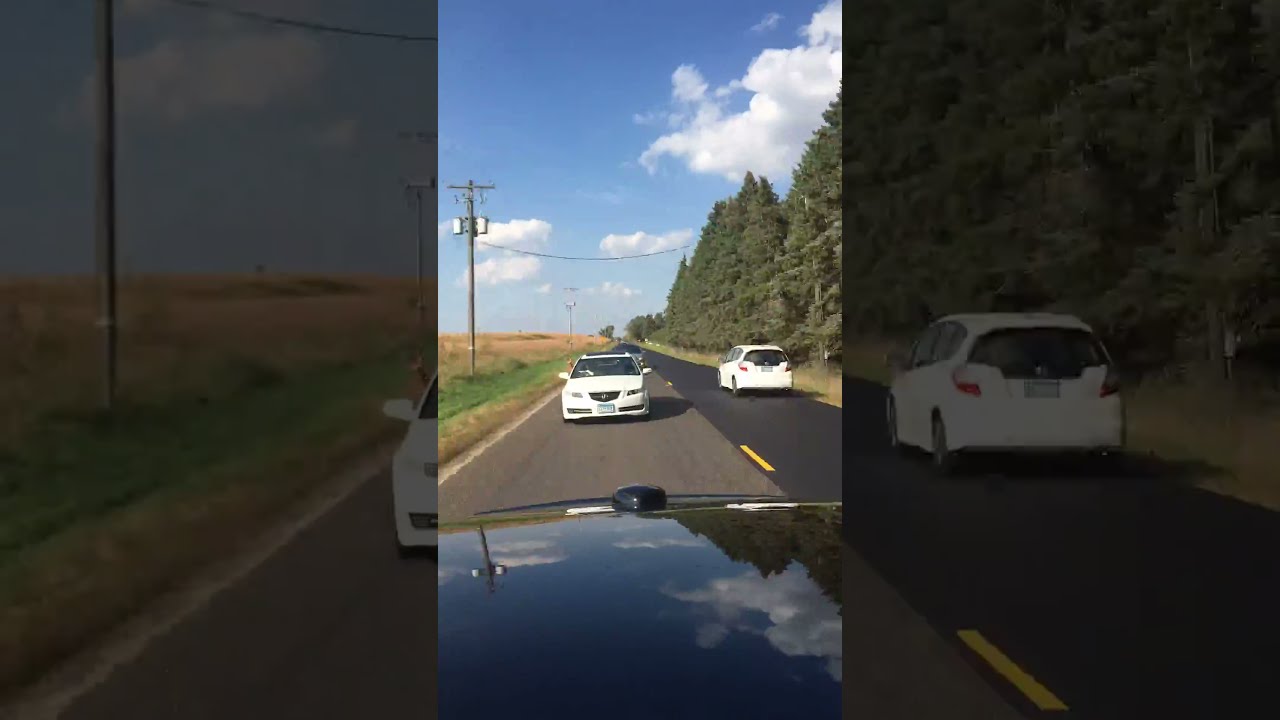The image is a vivid screenshot from a video, shown in a format where the middle part is clear while the sides are more muted, creating a focus effect. The scene captures the view through what seems to be the back of a dark or black car. The hood of this car reflects the sky, clouds, and trees vividly. In the center of the image, a shiny white car faces the viewer, hinting it's either approaching or stopped directly behind the dark car.

The surrounding road is a two-lane highway characterized by a dotted yellow line indicating a passing zone. On the right side of the road, a white van is moving away from the scene, disappearing into the distance. The pavement to the right is darker than the left side, possibly due to recent roadwork.

To the right of the road, there is an array of large green pine trees, while the left side features tan and green grass fields interrupted by telephone poles and wires. The background sky is a harmonious mix of partly cloudy and fully blue, dotted with large, puffy cumulus clouds. In the distant left background, a brown wheat field can be observed, adding depth to the overall landscape.